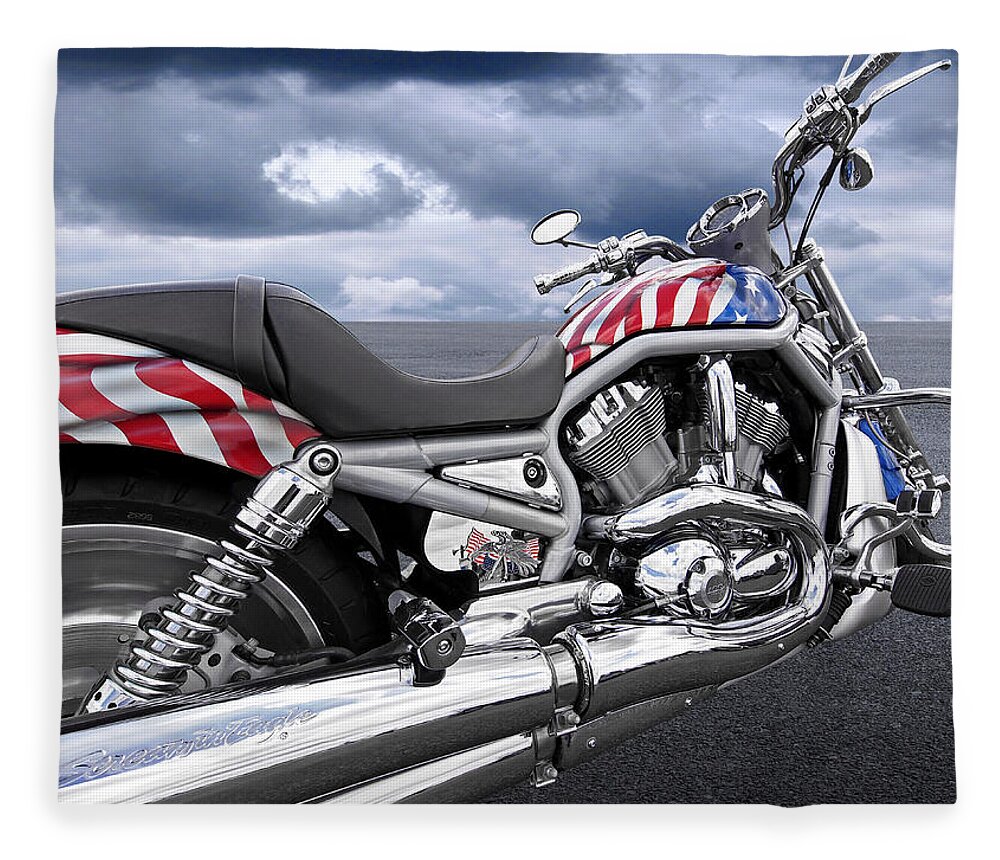This colored, close-up photograph captures a highly polished motorcycle standing on a vast expanse of asphalt that stretches to the horizon. The sky above is mostly covered with gray clouds, interspersed with darker blue areas that suggest a stormy atmosphere. The motorcycle boasts a custom paint job featuring vivid American flag designs with red and white stripes and a blue background with white stars; these details are prominently displayed on both the front hull and the rear fender. The chrome components shine brightly, including a notably curved chrome tube at the bottom left, the suspension system near the rear wheel, and the handlebars. The matte metal engine and custom components like the black leather seat with a distinctive sloping curve and possibly branded as "Serenity Eagle" add to the bike's uniqueness. The overall scene conveys an aura of rugged elegance against a backdrop of stark, open land.